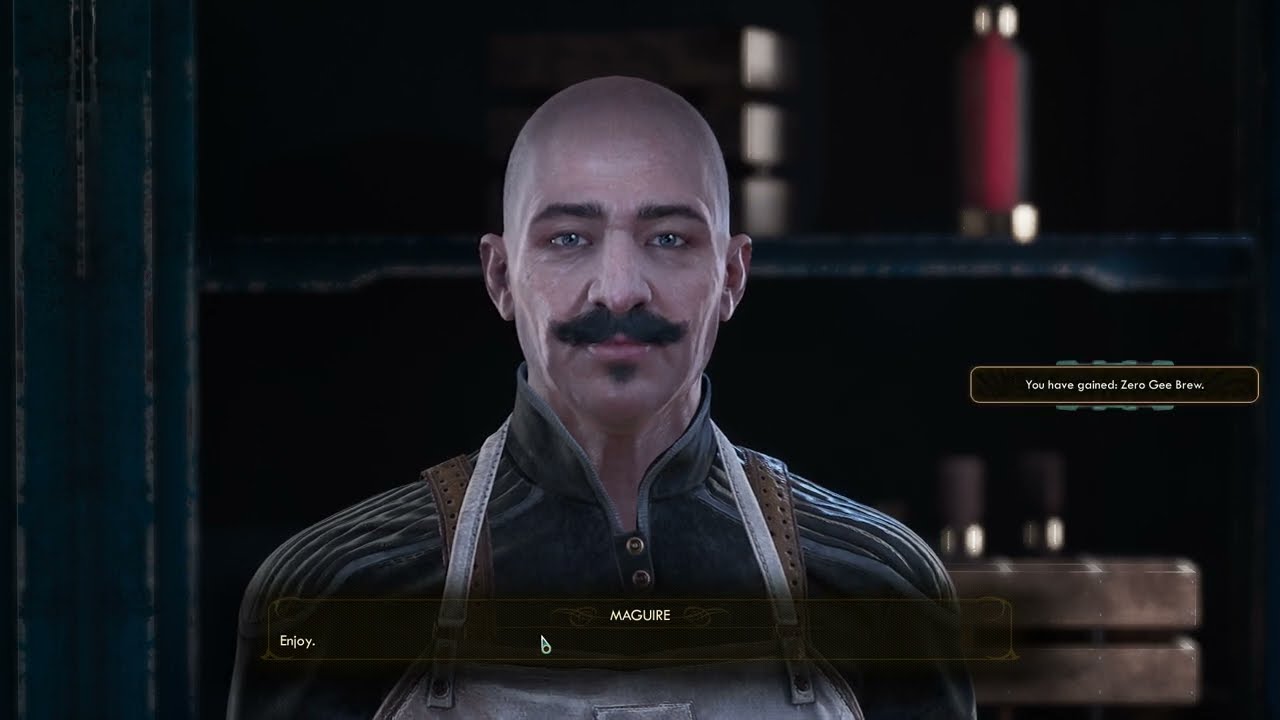The image is a detailed screenshot from a video game. It features a middle-aged, bald Asian man with a thick black mustache and a small black goatee, facing the camera with a neutral expression. He has black eyebrows, light skin with some wrinkles, and gray-blue eyes. The man is wearing a black striped shirt with gold buttons and a raised collar, with a white apron that bears the name "MAGUIRE" in white letters across his chest. 

The scene is slightly dim and blurry in the background, highlighting several items on shelving units behind the man. There’s a red thermos bottle at the top, and below it, several dark brown bottles with shiny silver tops and bottoms. A blue metal beam runs vertically to the left of the man, and on the lower right, there’s a visible box or crate. 

Text overlays the image: a transparent brown rectangle at the bottom shows "MAGUIRE" in white print, with “ENJOY” in the lower left corner, and another rectangle to the right reads "YOU HAVE GAINED 0GBREW" with "G" spelled out as "G-E-E".